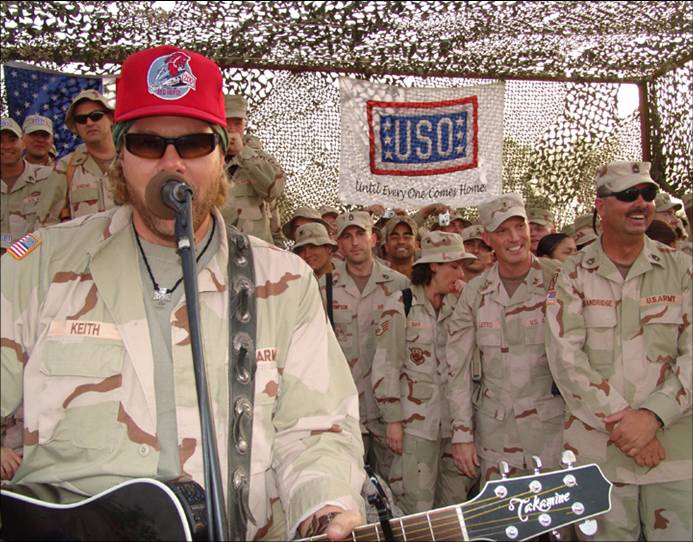This color photograph in landscape orientation captures a lively scene of over 20 U.S. Army soldiers. At the left side of the image stands the main subject, Keith, easily identifiable by his name tag and his distinct red hat. Keith is dressed in army fatigues and is engaged in an animated performance, playing an acoustic guitar and singing into a microphone. He accessorizes with a black leather string around his neck. To his right, a group of soldiers is gathered, some looking off to their left and laughing, while others focus on Keith’s performance with smiles on their faces.

In the background, a camouflage net drapes over the area, adding to the military ambiance. Prominently displayed is a flag featuring the U.S.O. logo, composed of a blue rectangle with six white stars framed by a red border, accompanied by the heartfelt slogan "Until Everyone Comes Home." An American flag is also visible, reinforcing the patriotic spirit of the scene. The photograph embodies representational realism, capturing a candid and heartwarming moment among the troops.